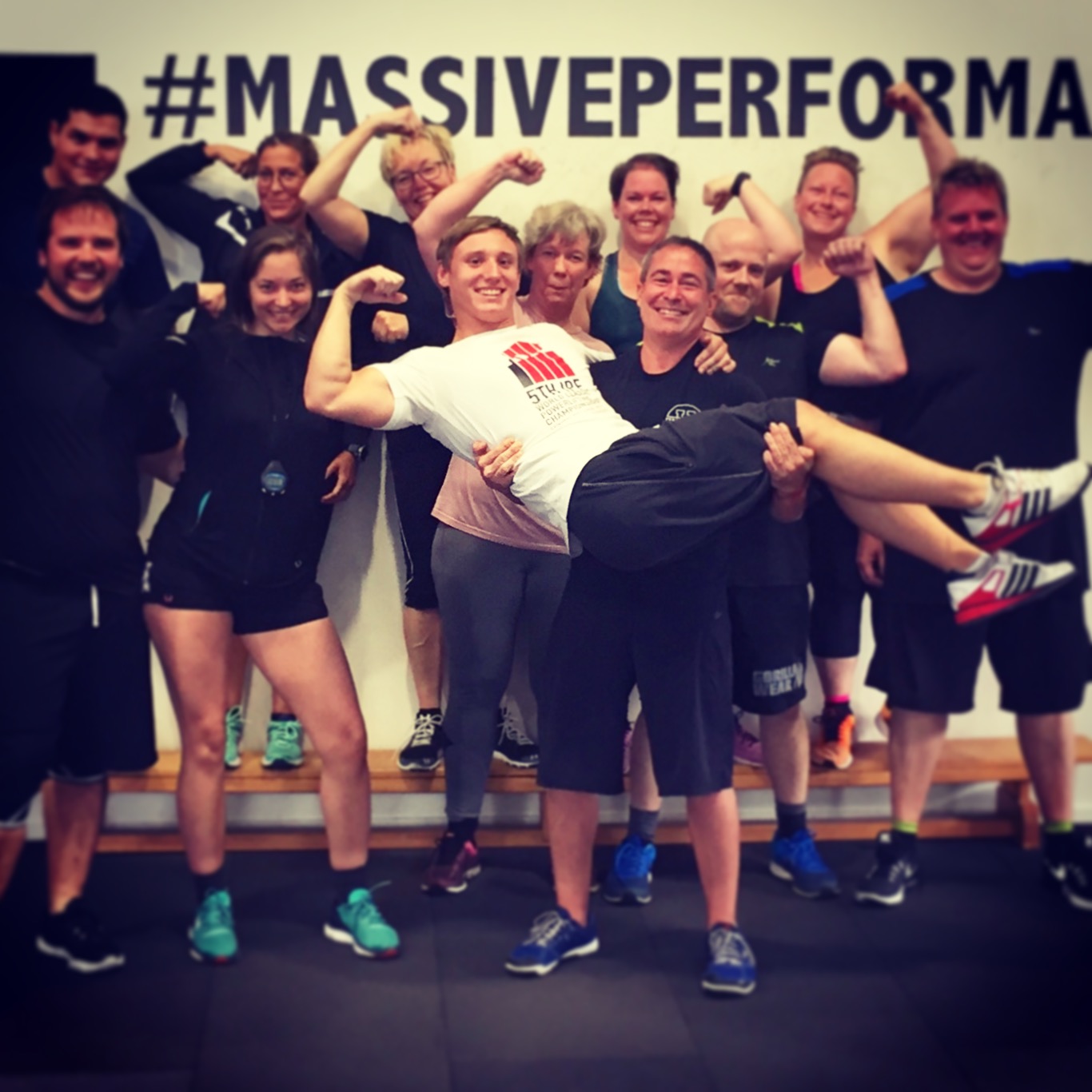In this energetic and joyful photo, a diverse group of around 10 to 15 fit and smiling individuals, likely athletes or gym-goers, are proudly flexing their muscles. Central to the scene, a muscular man in a white shirt with a red and blue design, paired with black shorts, is being held cradle-style by another very strong man who, although not flexing due to his occupied arms, exudes strength. Most individuals are dressed in black attire, with the notable exceptions of the man in white and a woman situated towards the center-back, wearing a light pink shirt. The backdrop features a partially visible hashtag that reads "#massiveperform," hinting at the full word "performance." The group exudes happiness and camaraderie, with everyone, young and older alike, showing enthusiasm and athletic spirit as they proudly display their impressive physiques. The scene is filled with energy and unity, underscored by the varying yet complementary lengths of their black shorts and their uniform footwear.